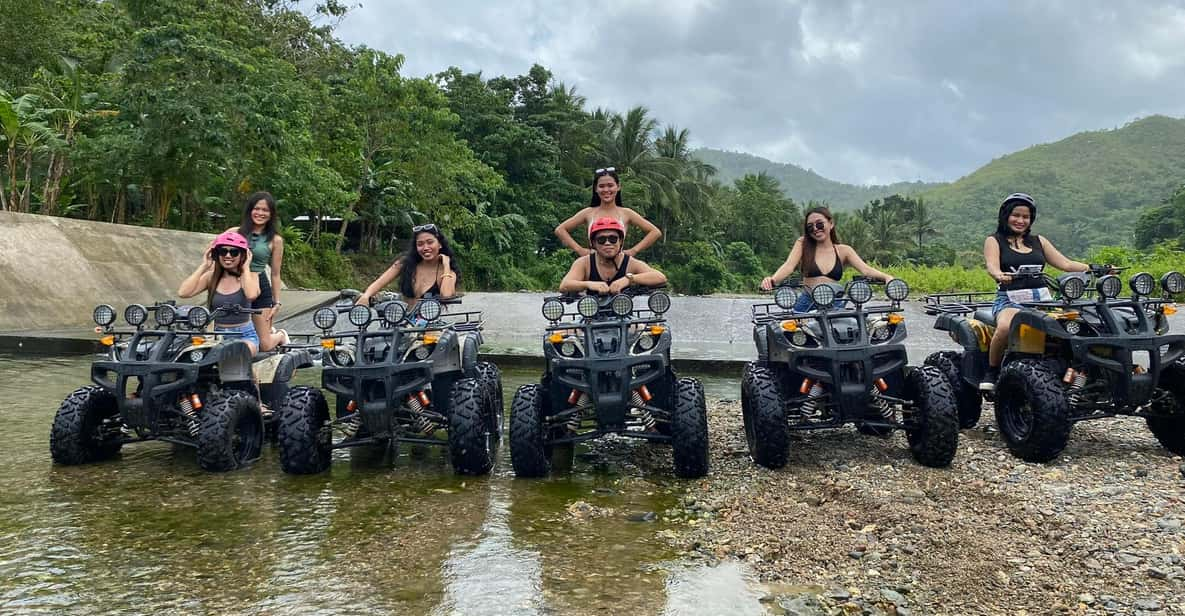The image showcases a dynamic scene of seven individuals navigating rugged terrain in ATV-like vehicles within a marshy, jungle area. The group consists predominantly of women; three are seen riding their vehicles solo, while a few are paired up on the remaining ATVs—two women on one and a man with a woman on another. The vehicles, designed for challenging environments, confirm their utility with large, all-terrain tires and multiple headlights. They appear to be traversing a puddle-strewn, rocky riverbed, contributing to the sense of adventure. Surrounding the group is a lush landscape featuring dense, green tropical foliage and palm trees, set against the backdrop of distant, verdant mountains under an overcast sky. The riders, seemingly triumphant, smile at the camera, capturing a moment of shared accomplishment.